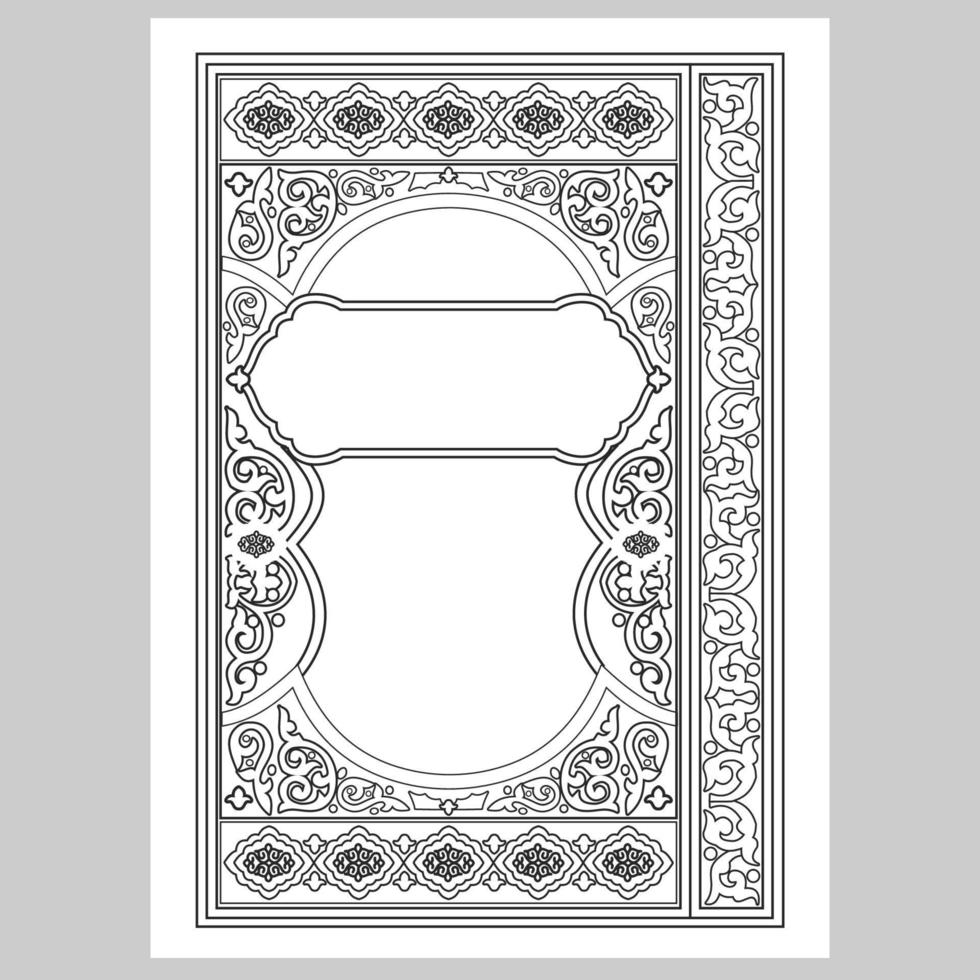The image is a black and white design with a gray background, resembling a book cover or a decorative card. The design is printed on a white rectangular sheet of paper, which is framed by a thick gray border on the sides and thinner gray lines at the top and bottom. The design incorporates various intricate patterns, including curved shapes and ornamental motifs reminiscent of old book or manuscript decorations.

Around the central blank space, which is likely intended for a title or an author’s name, there are two black lines bordering it. The central blank area is flanked by repeating decorative elements. On the right side, there are patterns that resemble opposing 'G' shapes or leaves, interspersed with dots, and this motif recurs vertically. The top and bottom sections of the main rectangle also showcase a floral design interspersed with repeating plus symbols.

These ornate patterns create a symmetrical and repetitive design that wraps around the central blank area, adding a classic and ornamental touch to the sheet. Overall, the detailed black motifs against the white paper, framed by the gray background, give the impression of an elegantly designed book cover or an ornate document.